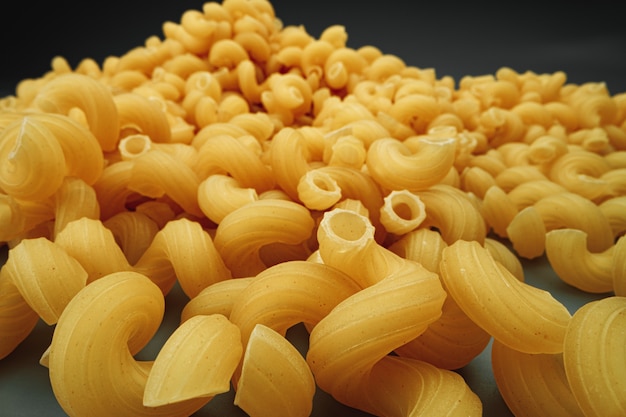The image showcases a pile of uncooked Cavatelli pasta against a dark gray background with a blue-gray surface. The pasta noodles are bright yellow with a slight orange hue, and they are shaped in a unique spiral form with grooves along their length, reminiscent of a helix. Some noodles are visibly hollow at their ends, adding to the intricate texture. The Cavatelli are bunched up in the rear center-left of the image, creating a visually striking contrast with the dark background. Overhead lighting brings out the details in the twisted, tubular shapes of the pasta, emphasizing their distinctive appearance.